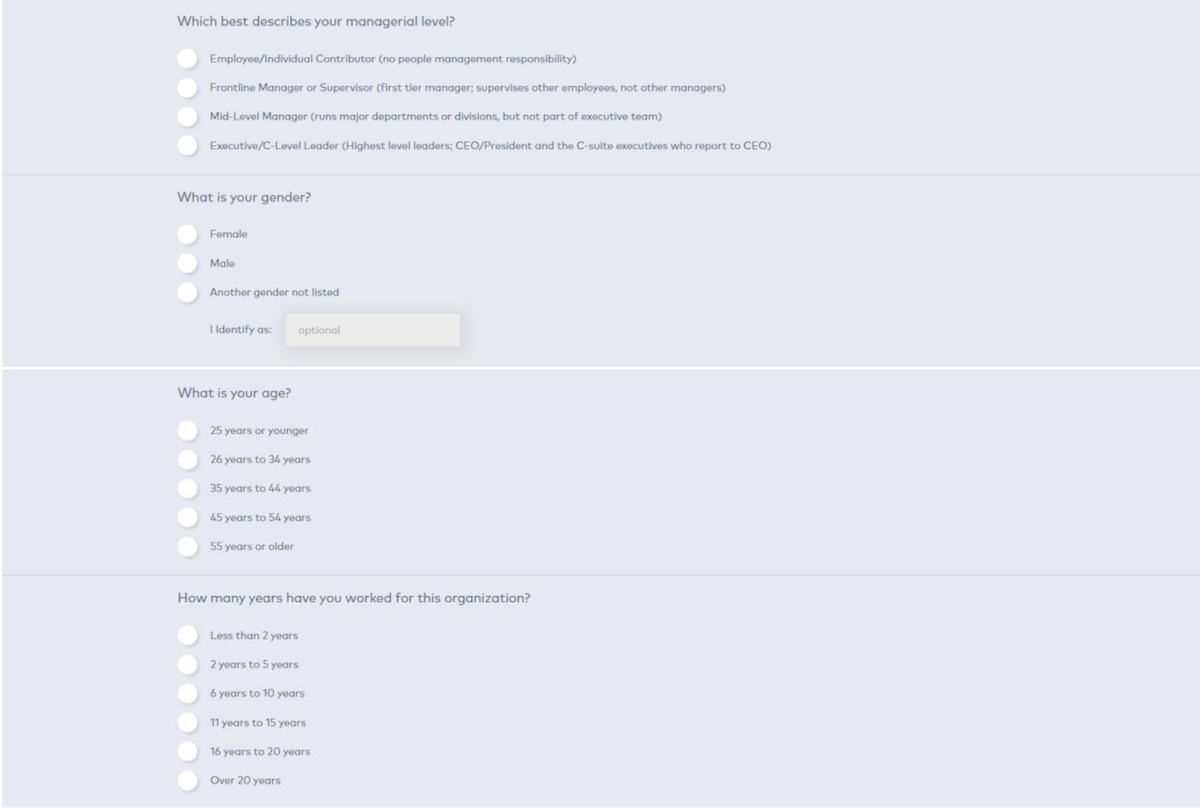The image displays a survey form with multiple-choice questions designed to gather information about the respondent's managerial level and gender. The form has a light gray background, and each question is accompanied by response options that can be selected via white circles to the left of each choice. 

The form is divided by a distinct white line that horizontally separates the second and third questions. 

1. **Question about Managerial Level:** "Which best describes your managerial level?" 
   - **Options:**
     - Employee (Individual contributor, no people management responsibility)
     - Frontline Manager or Supervisor (First-tier manager or supervisor)
     - Mid-Level Manager (Runs major departments or divisions but not part of an executive team)
     - Executive (C-level leader, highest level leader such as CFO, President, in the C-suite reporting to CEOs)

2. **Question about Gender:** "What is your gender?"
   - **Options:**
     - Female
     - Male
     - Another gender not listed